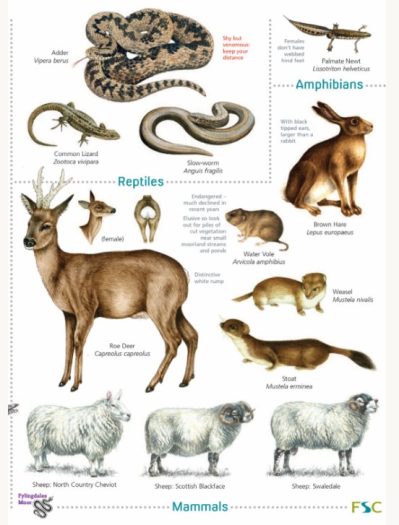The image features a white background and is formatted in a portrait layout, meaning the height is shorter than the width. It is sectioned off into three labeled categories: reptiles, amphibians, and mammals. In the top-left section titled "Reptiles" (in blue text), there are detailed pictures of two different snakes, a slow worm, and a lizard, each with descriptive text beneath them. On the top-right, under the label "Amphibians" (also in blue text), there is an image of a pale mate newt with small, somewhat blurry text below it. The bottom section is dedicated to "Mammals" (again written in blue text) and depicts a variety of animals including a deer, a brown hare (which is a type of rabbit), a water vole, a weasel, and a stoat. Clearly visible in this section are a deer head and a partial view of a deer tail. Additionally, there are three kinds of sheep, colored in shades of white, while the remaining mammals such as the deer, rabbit, mouse, and otter-like animal appear in various shades of brown. The edges of the image feature logos in the lower right and lower left corners. Overall, the lighting is bright and the animal illustrations are clear, although the accompanying text is small and somewhat blurry.